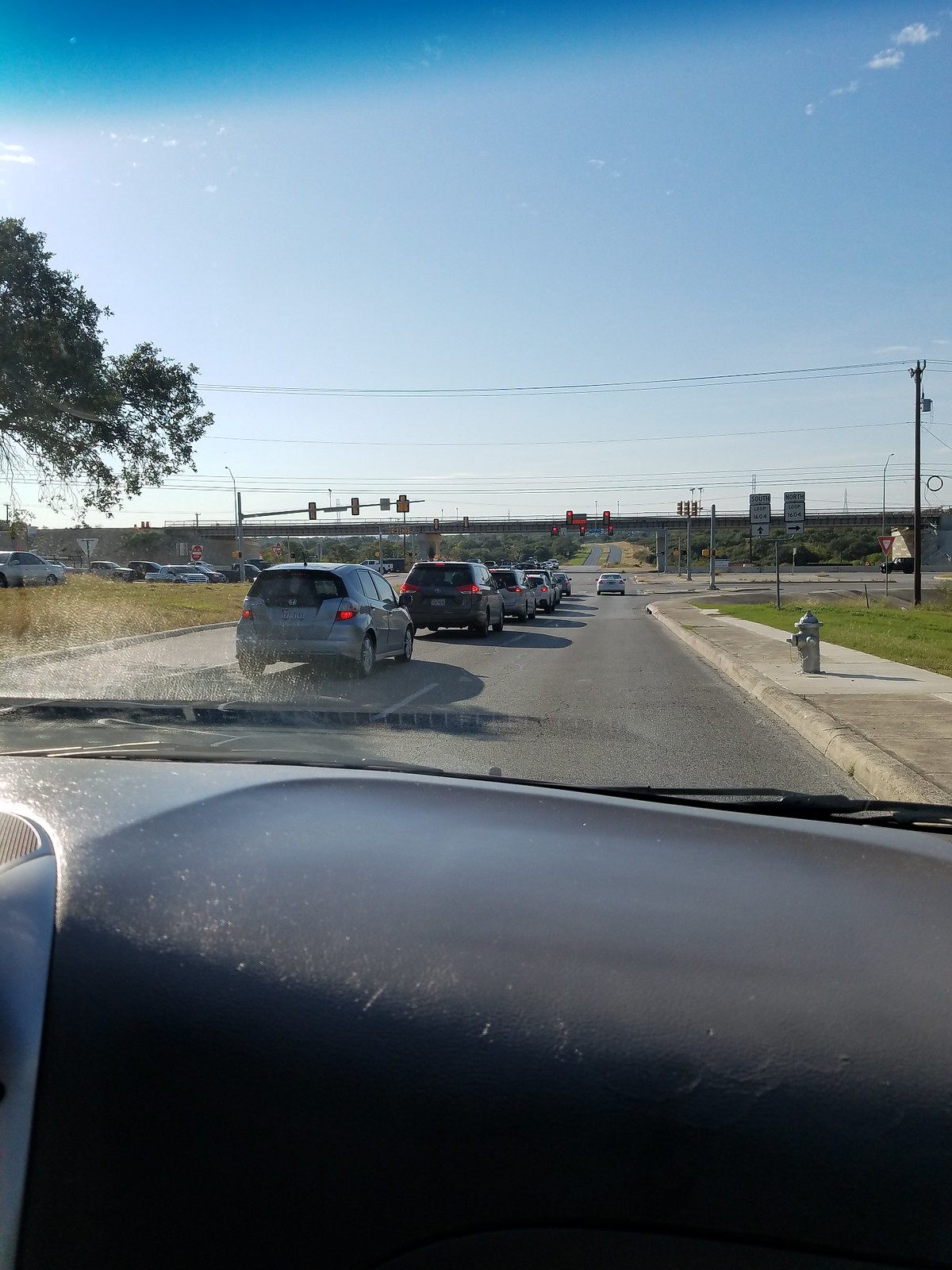The photograph, taken from inside a car, presents a scene through the slightly dusty black plastic dashboard. In the reflection of the windshield, air vents are visible, with the car's wiper also in sight just above the dashboard. Outside the car, the left lane is occupied by five vehicles, while one car is positioned directly ahead. The left side of the image shows dry grassy fields and the upper part of a tree with green leaves. Electrical lines stretch across the middle of the image, and a utility pole stands on the right. On the right-hand side, there's a green grassy area, a sidewalk, and a blue fire hydrant. The sky above is a deep blue with scattered white clouds.